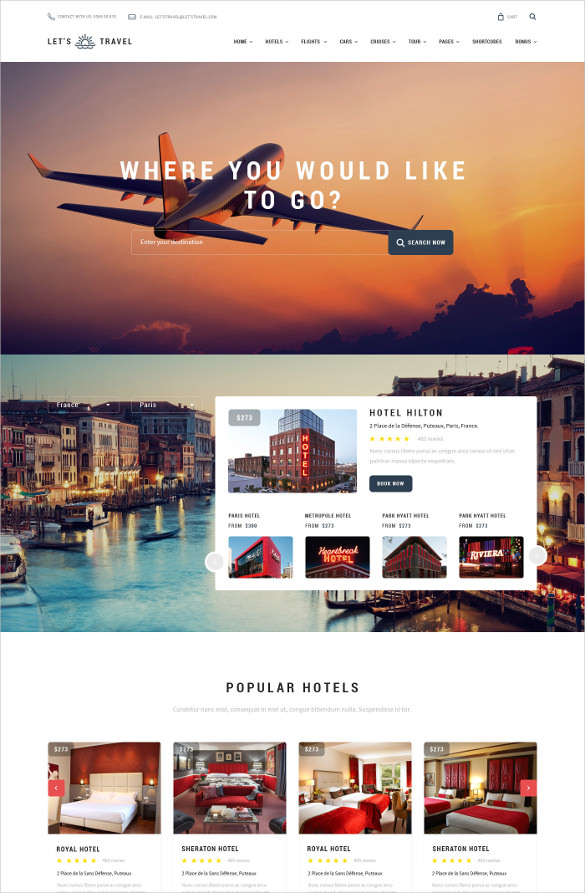This screenshot is taken from a luxury travel website named "Let's Travel." The website offers users the ability to book flights to various global destinations and settle into hotels at their holiday locations. The interface prominently displays hotel options, starting with Hotel Hilton, which is available for booking. Other notable hotels listed include the Paris Hotel, the Metropolis Hotel, and the Parcouillat Hotel.

At the bottom of the page, there's a selection of popular establishments such as the Royal Hotel and the Sheraton Hotel. These hotels are shown with their respective prices, which are quite high, for example, $273 and $213 per night, indicating a high-end market. Each hotel listing includes a star rating, with all displayed options boasting a 5-star rating.

The website features a luxurious design, highlighted by its elegant logo "Let's Travel," which is situated above a clearly displayed phone number for customer inquiries. Additionally, the site offers various interfaces for customers to communicate with travel agents.

Dominating the center of the screen is an image of a plane soaring towards a tropical destination, adding to the aspirational and premium feel of the website.